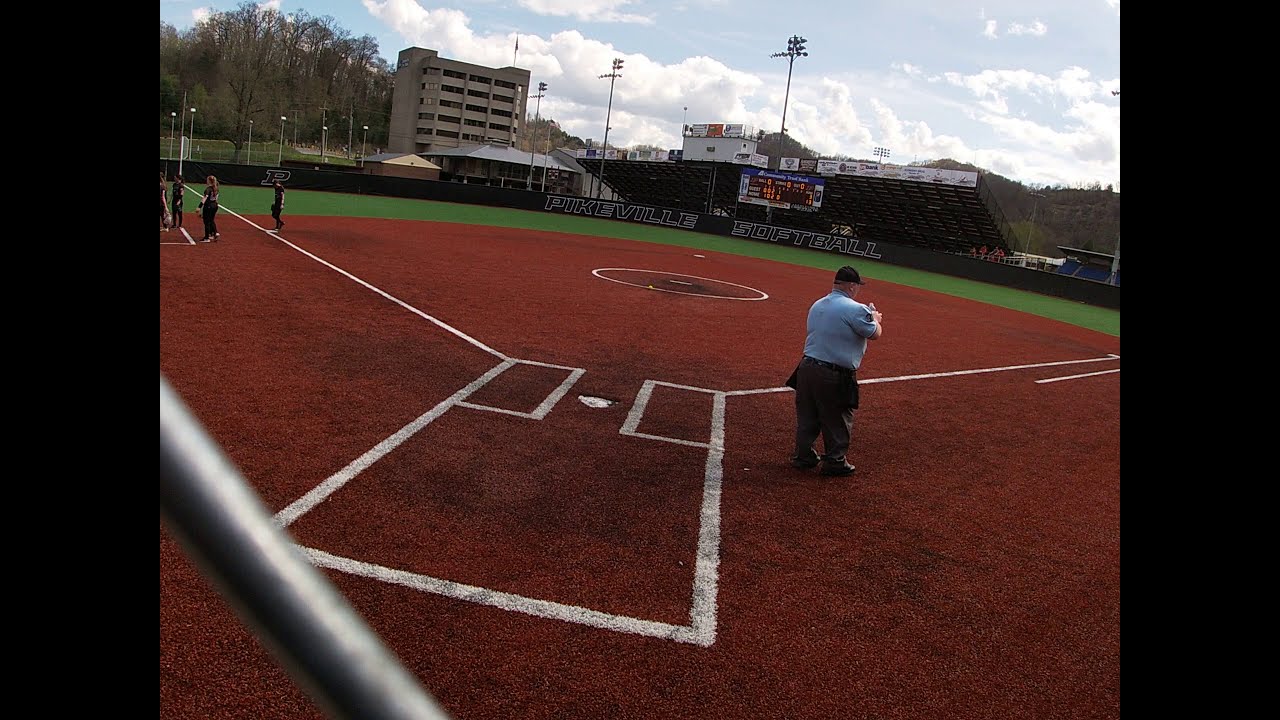The photograph depicts an expansive baseball field characterized by its predominantly empty and serene atmosphere. At the heart of the field, an older, heavyset gentleman stands with his back towards the camera, dressed in a blue shirt, brown or possibly gray pants, and a black cap. The field itself is a striking red with detailed white line markings, bordered by a narrow strip of vivid green grass near the boundary.

On the left side of the field, a small group of sports girls can be seen standing in the distance, hinting at recent or imminent activity. The boundary fence prominently displays the words "Pikeville Softball," adding to the venue's identity. Beyond the boundary, there's a variety of background elements including spectator bleachers, a multi-story building, and some lush green trees. A prominently placed scoreboard and elevated stadium lights enhance the field’s ambiance, while the bright blue sky dotted with white clouds offers a picturesque backdrop. Adding to the details, a silver metal pole is noticeable in the front left-hand corner of the image.